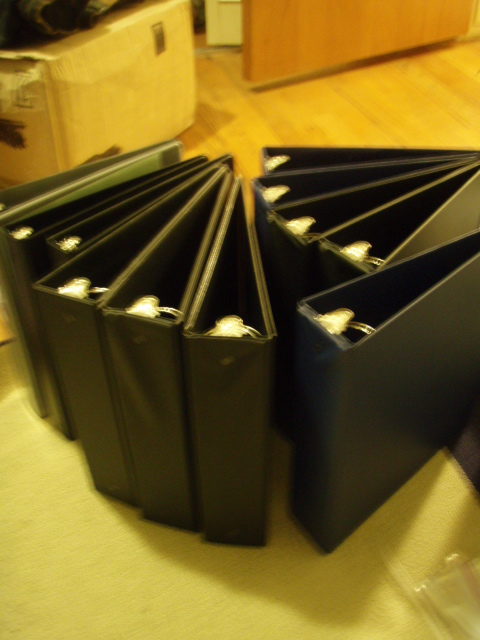In this blurry, out-of-focus photograph taken indoors in portrait mode, a collection of empty loose-leaf binders is prominently displayed in the foreground. There are approximately 12 binders, predominantly black, with one navy blue binder among them. Seven of the binders are arranged side by side on a white desk to the left, forming a triangular wedge due to their close arrangement. To the right of these, five additional black binders are similarly grouped, with their edges pointing outward to the left of the frame. The tops of the binders reveal silver rings meant for holding papers.

In the background, the floor features dark brown and orange woodgrain, extending towards a wooden door, whose bottom and the shadow beneath it are visible. In the upper left-hand corner of the image, a slightly open door is also seen, while next to it sits a light brown cardboard box with some dark items—possibly green—on top of it. The lighting in the room casts a yellowish tint over the scene, contributing to the overall blur and soft focus of the image.